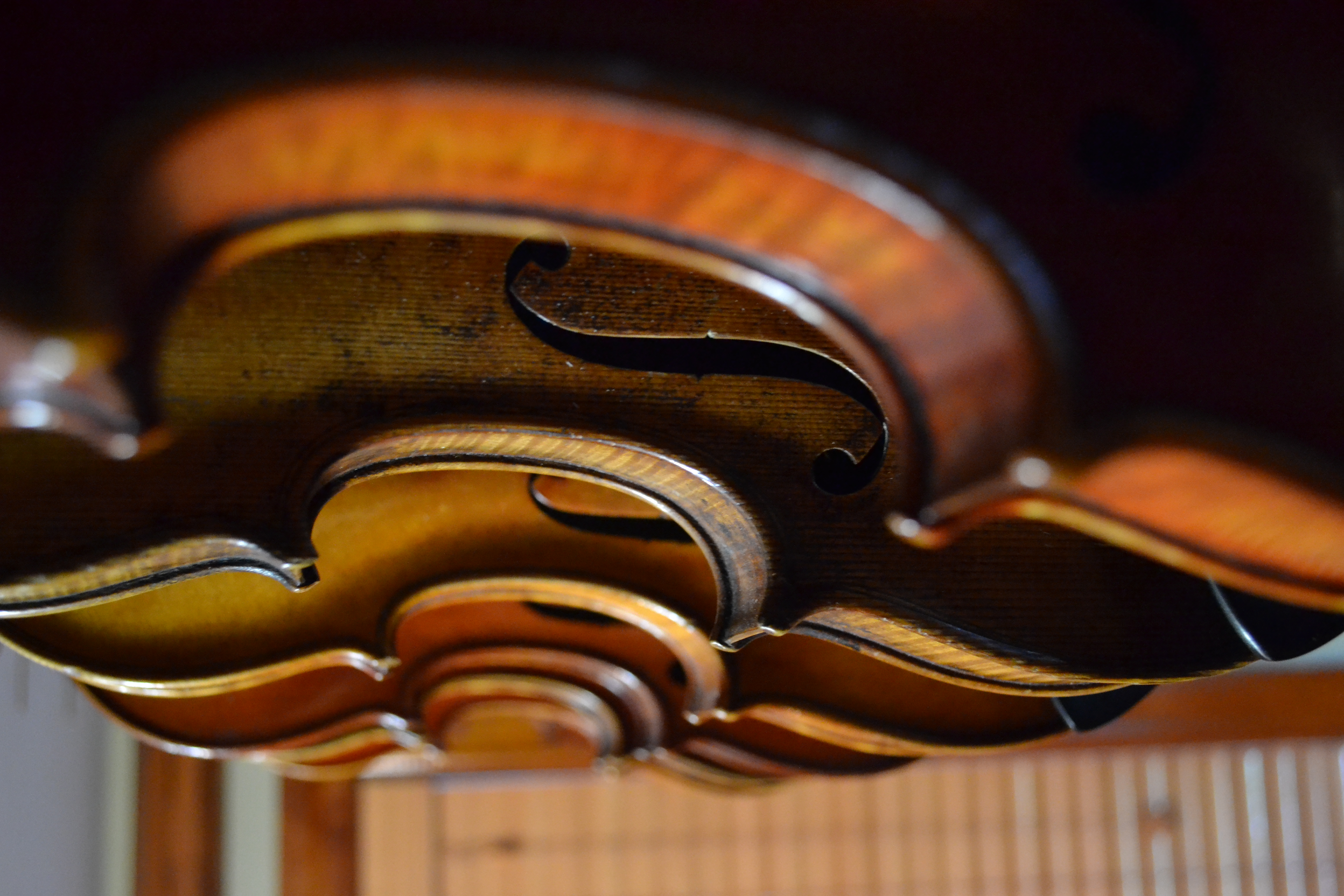This photograph features an extremely zoomed-in, close-up view of an intricately carved wooden object, possibly part of a musical instrument such as a violin, cello, or bass, or an elaborately adorned piece of furniture. The main subject is a richly polished, golden-brown wood, showcasing fine details of varying wood grain and multiple layers of thin, petal-like wooden elements arranged vertically. Centrally, a round wooden piece unifies the entire structure. Prominently featured within the composition is a distinctive black metal S-shaped figure, resembling a musical symbol, potentially adding resonance or aesthetic flair. The background is purposefully blurred, consisting of light-colored wooden slats of a paneled wall, adding depth to the image. The top portion of the photograph fades into total darkness, making the foreground details stand out sharply.